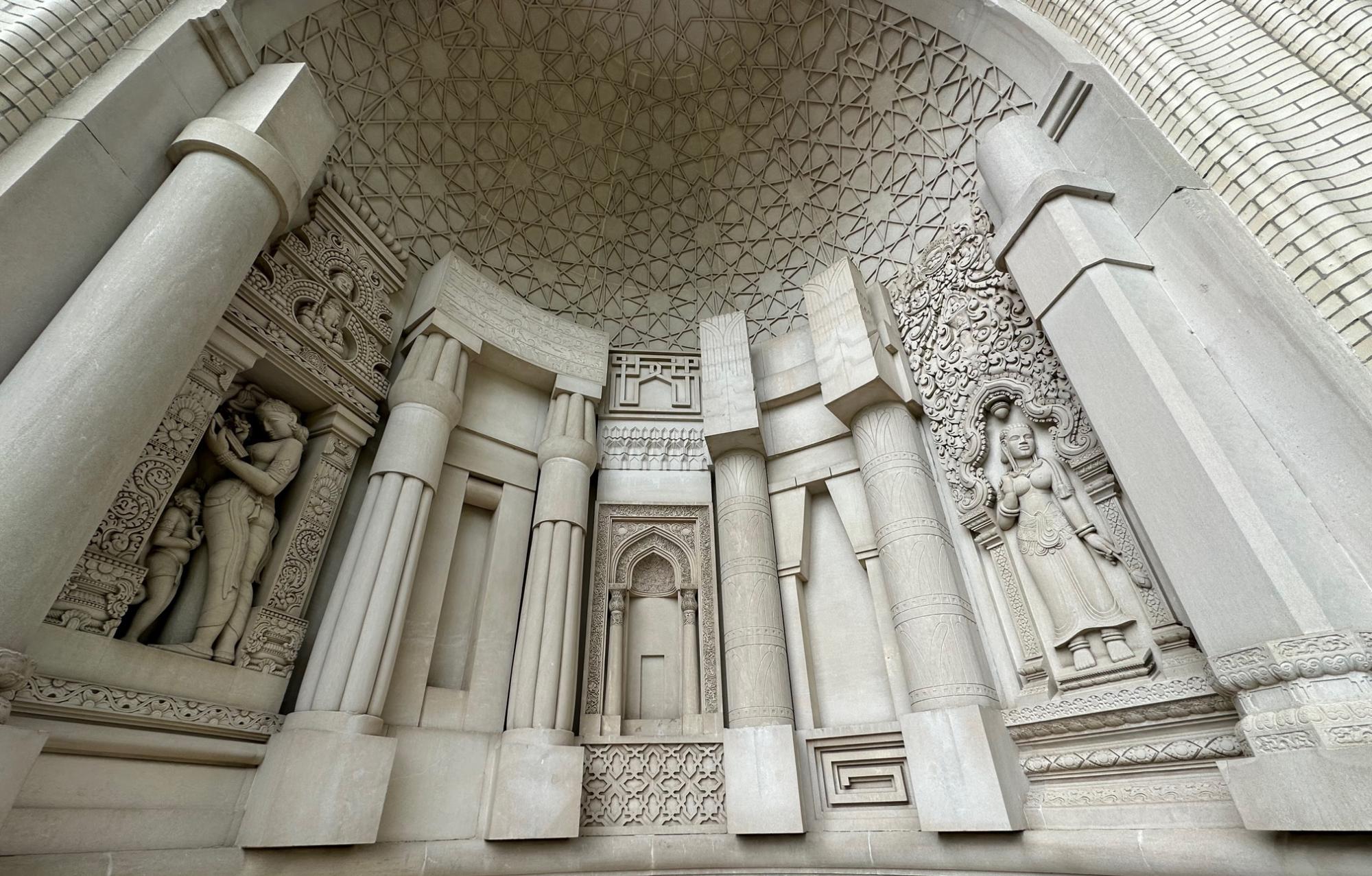This color photograph captures the grandeur of a very ornate interior, likely belonging to a grand cathedral or museum, designed in a style reminiscent of Greek or Roman architecture. Taken with a wide-angle lens, the photograph emphasizes the curvature and vastness of the space, focusing on the intricately carved, domed ceiling. The room is dominated by tall, imposing granite and marble columns that ascend towards the ceiling, each uniquely styled with ornate patterns and carvings along their bases and surfaces. 

Prominently featured within the columns are two distinctive figures— on one side, an older person stands with a child beside them, both figures carrying staffs and rendered in intricate 3D-like carvings, as though they have been etched into the stone itself. On the opposite side, a similar level of detail reveals a young woman with long hair, standing protectively over what appears to be a church, illustrating a sense of watchfulness.

The color of the stone, an off-white or grayish-white akin to that of the White House, enriches the regal aesthetic, complemented by mosaics of triangular tiles adorning the ceiling, adding further complexity to the patterning. Additionally, artwork integrated into the walls shows a young girl reading to a young boy, perhaps searching through a book for a recipe or information, enhancing the narrative depth of the space. The overall impression is one of magnificence and historic reverence, capturing the essence of the building's architectural and artistic opulence.